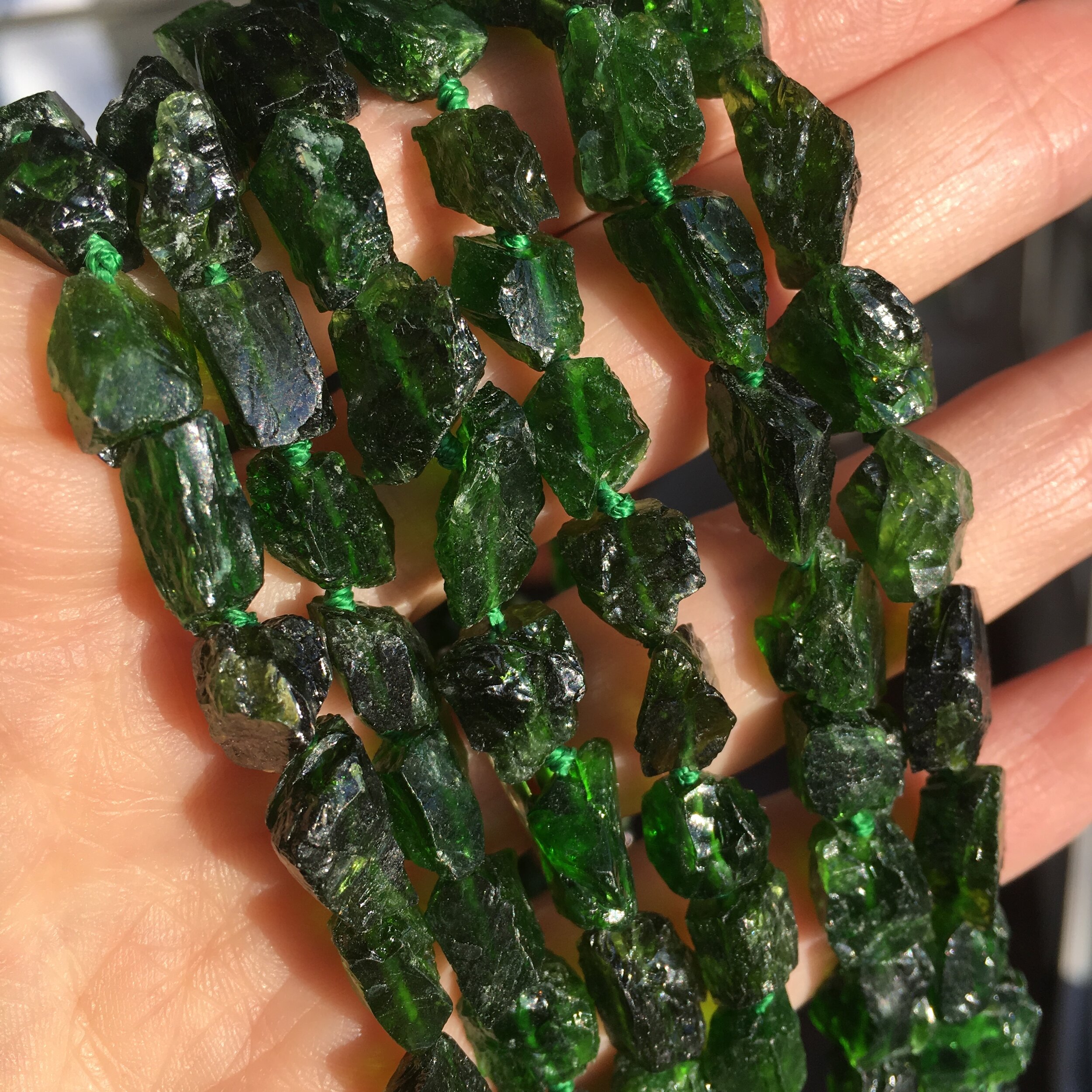This close-up image showcases a piece of rock jewelry, specifically a green necklace, displayed across the fingers and upper palm of a white hand. The necklace features six lines of rough-cut emerald stones, each separated by green knots of fabric, creating a harmonious yet rugged aesthetic. The stones display varying shapes and sizes but remain relatively uniform in their jagged form. They exhibit different shades of green, from dark to light, with some beads appearing almost translucent where the bright lighting hits them. The stones appear dusty and hard, resembling rough natural formations rather than polished gems. A faint white string runs through the stones, helping to keep this intriguing piece together. A light shadow is cast in the upper left corner of the image, adding depth to the detailed and brightly lit scene.